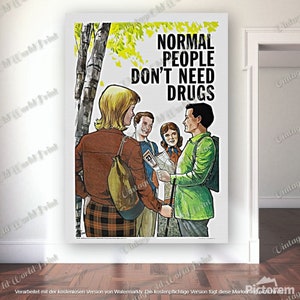The image displays a large, prominent poster hanging on a white wall, adjacent to a doorway and above dark hardwood flooring. The poster nearly spans the entire height of the wall and features bold black text, all in capital letters, in the upper right corner that reads: "NORMAL PEOPLE DON'T NEED DRUGS." Below the text, a cartoon illustration of four individuals is depicted. One character is a blonde person wearing a brown jacket. Next to them stands a white male with short brown hair in a blue sweater. Another individual, a woman with short brown hair, is dressed in a brown button-down shirt and a white vest. The final character is a man with black hair donning a bright green jacket and carrying a backpack. They are positioned near the trunk of a tree with lime green leaves. The overall scene gives the impression of being displayed in a home setting.